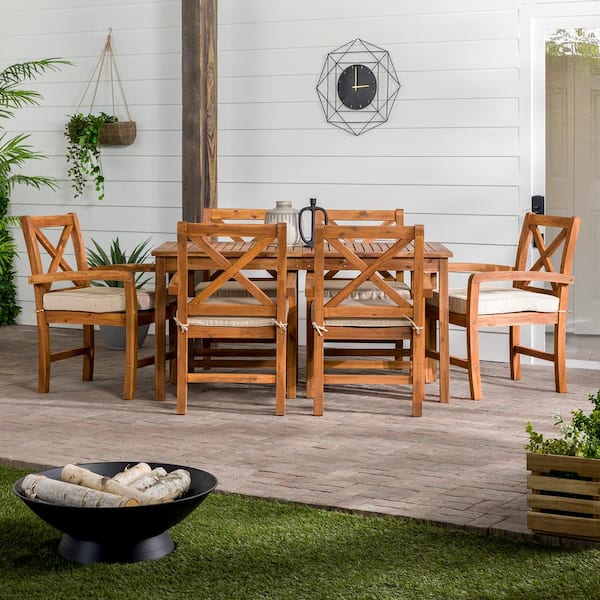The photograph depicts a meticulously staged outdoor scene that was likely captured in a photo studio, as evidenced by the artificial grass and lighting. At the forefront, there is a small black fire pit filled with white birch logs, placed on clearly synthetic grass. The scene centers around a medium-brown wooden table surrounded by six matching chairs. Each chair has a beige cushion securely tied to it, arranged symmetrically with two on each side of the table and one at each end, all positioned on a brick patio. In the middle of the table, there is an object resembling a lamp with its lampshade resting on the tabletop. The backdrop features a white clapboard house adorned with a distinctive modern clock showing 3 o'clock, and a hanging peat basket planter with cascading ivy on the left side. A doorway is partially visible to the right of the clock, enhancing the homely atmosphere of the setting. Green foliage peeks out from the left, adding a touch of natural flair to the otherwise artificial environment.